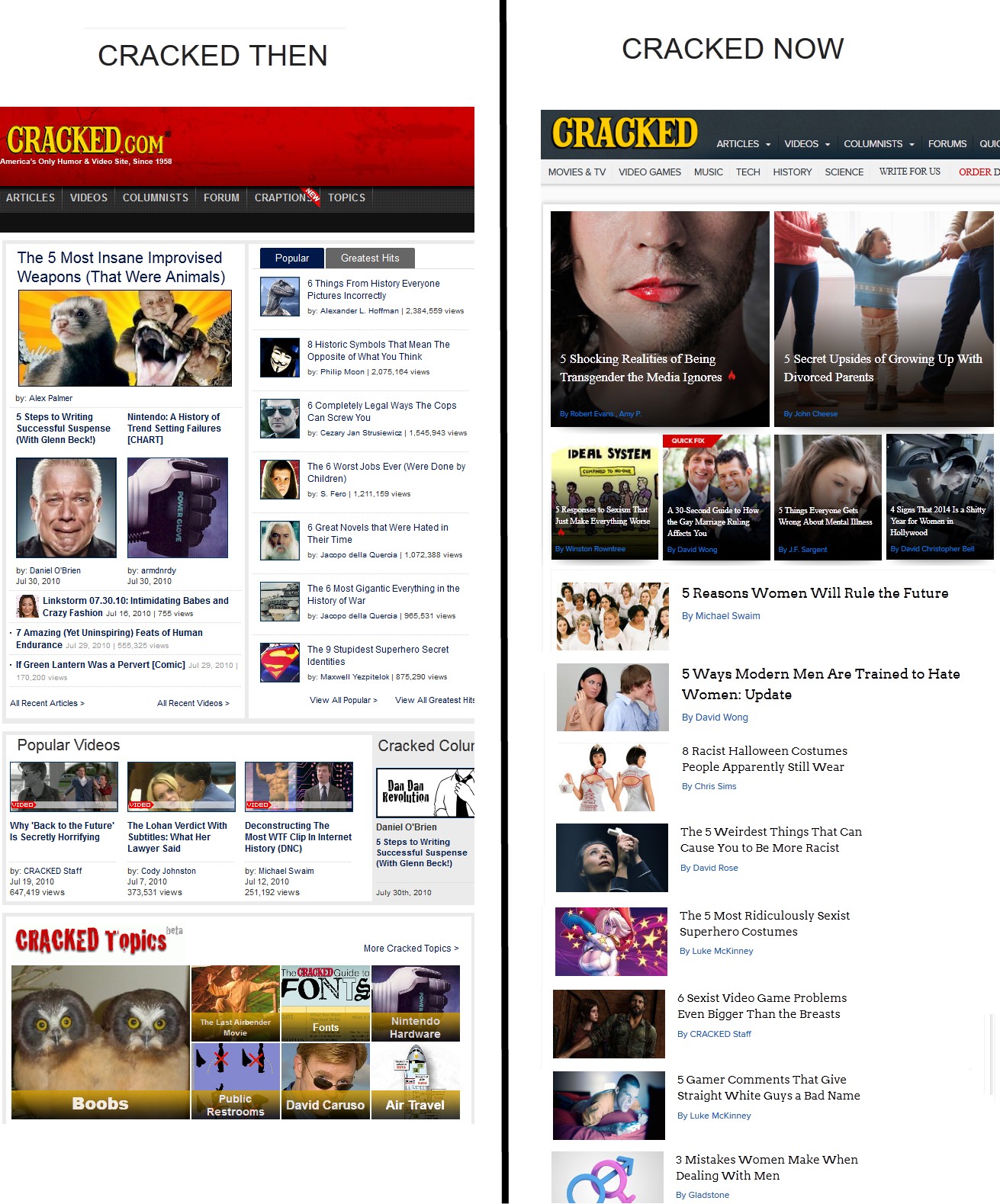A split-screen screenshot juxtaposes two iterations of the Cracked.com website. On the left, the older version of the site features a bold red header with yellow text, proclaiming "Cracked.com" and beneath it, in white text, the tagline "America's only humor and video site since 1958." Directly below, a gray navigation bar with white text lists sections from left to right: Articles, Videos, Columnists, Forum, Craptions, and Topics. A distinct red banner with white text reading "New" runs diagonally across this header. The main article showcased is titled "The Five Most Insane Improvised Weapons (That Were Animals)," accompanied by an image depicting a ferret, a cobra, and a baby set against a vibrant yellow and orange background.

The right side of the screenshot features the modern version of Cracked.com, labeled "Cracked Now" at the top. This version has a sleek gray header with yellow text simply reading "Cracked." To the right, the sections listed are Articles, Videos, Columnists, and Forums. Below this primary navigation, additional categories are presented in black text on a gray background: Movies and TV, Video Games, Music, Tech, History, Science, Write for Us, and Order.